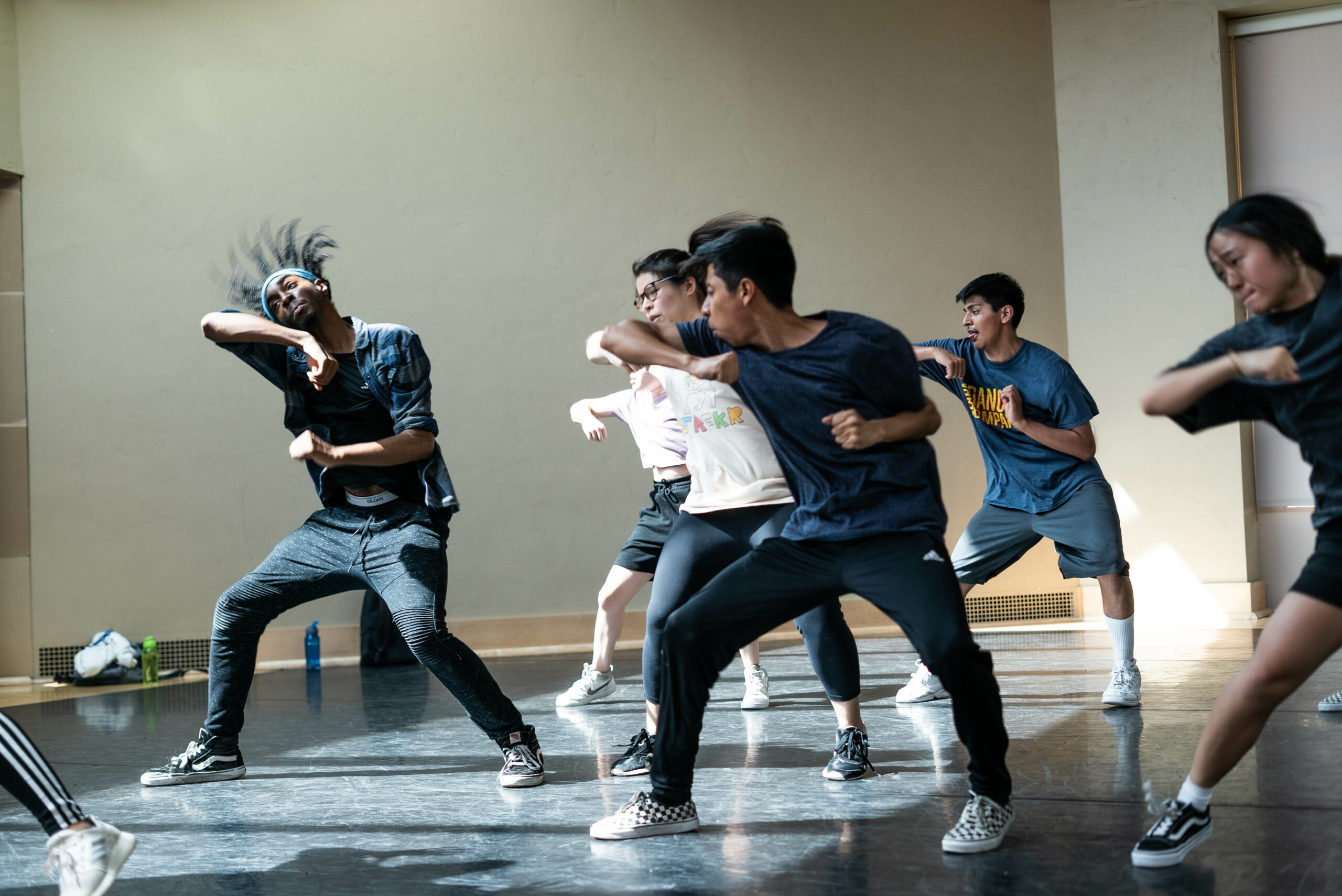In a sunlit dance studio with beige walls and a black floor, a diverse group of six dancers are captured mid-routine. Beams of sunlight cast across the floor from unseen windows, illuminating the dancers' synchronized movements. They all have their right elbows extended, hands curled towards their chests, and right feet out, their bodies slightly scrunched down in focused exertion. Among them, an African-American man with a blue headband, dark pants, and a blue top stands out on the left. To his right, some Asian dancers can be seen, including a man in a dark blue shirt and black pants. On the far right, a woman with black hair in dark sportswear completes the formation. Their dynamic poses are emphasized by the visible motion, such as the flying hair of the African-American dancer. The background reveals towels and water bottles neatly set up, indicating a well-prepared practice environment, as the dancers work hard in their comfortable, loose-fitting clothing and sneakers.